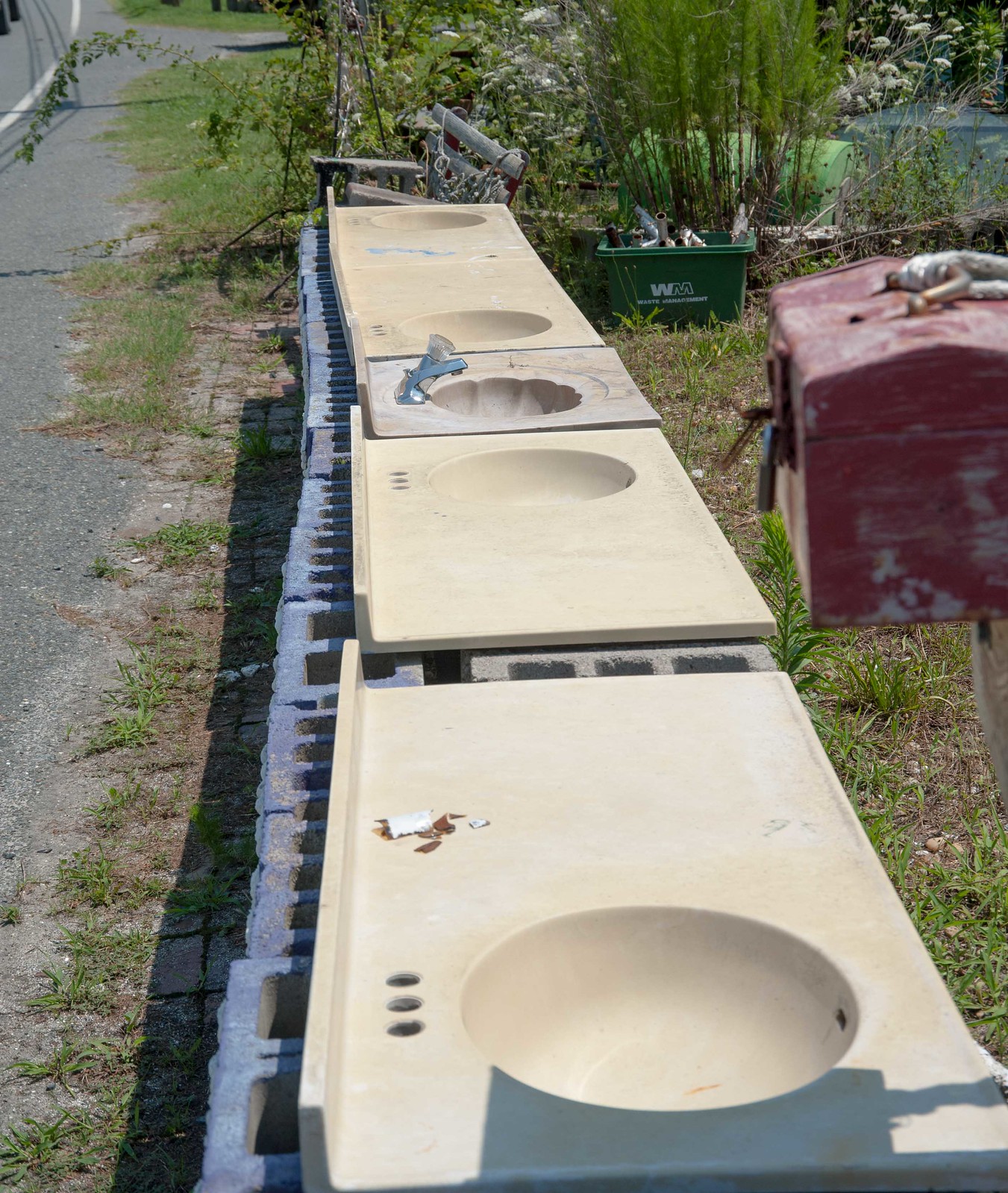The image depicts a row of outdoor bathroom sink countertops placed on a long surface made from stacked gray cinder blocks, situated along the side of a road without a curb in a rural area. There are five sink countertops in total, with varying sink placements and colors. The closest countertop to the viewer has its sink on the left side, while the one next to it has its sink on the right. The middle countertop, smaller and distinct with a seashell-shaped sink and an attached faucet handle, is positioned centrally. The following two countertops alternate their sink positions, one on the left and the other on the right. The countertops are predominantly in off-white, beige hues, except for the middle one which has a marble-like appearance. 

In the background, there is an overgrown area with green weeds and grass, together with some planted shrubs. A green waste management bin, filled with pipe parts, is also visible. To the right of the countertops, a red, weathered chest or mailbox with a metal handle can be seen. The left side of the image shows part of the road surface with grass and dirt encroaching onto it.